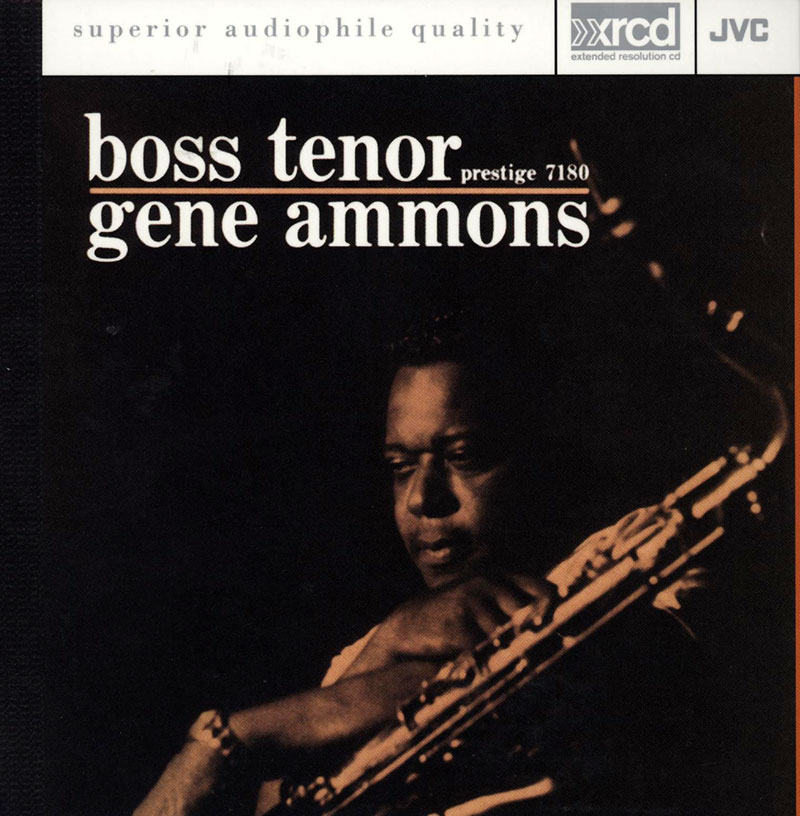The image is a detailed CD cover featuring a black man, identified as Gene Ammons, holding a saxophone. The man, who has dark skin and is wearing a watch on his left wrist, is depicted chest up and is staring towards the bottom left corner. He holds the saxophone with his right hand, which is positioned at an angle. The entire photograph is set against a very dark black background. The image is square-shaped, and the style is a high-quality, realistic photograph.

At the top of the cover, there is a banner reading "Superior Audiophile Quality, XRCD, JVC, Extended Resolution CD." Below this, the title "Boss Tenor, Prestige 7180" is prominently displayed. Beneath this title is the text "Gene Ammons." Additionally, the color palette of the image includes black, white, gold, brown, beige, and gray tones, contributing to its sophisticated and polished aesthetic.